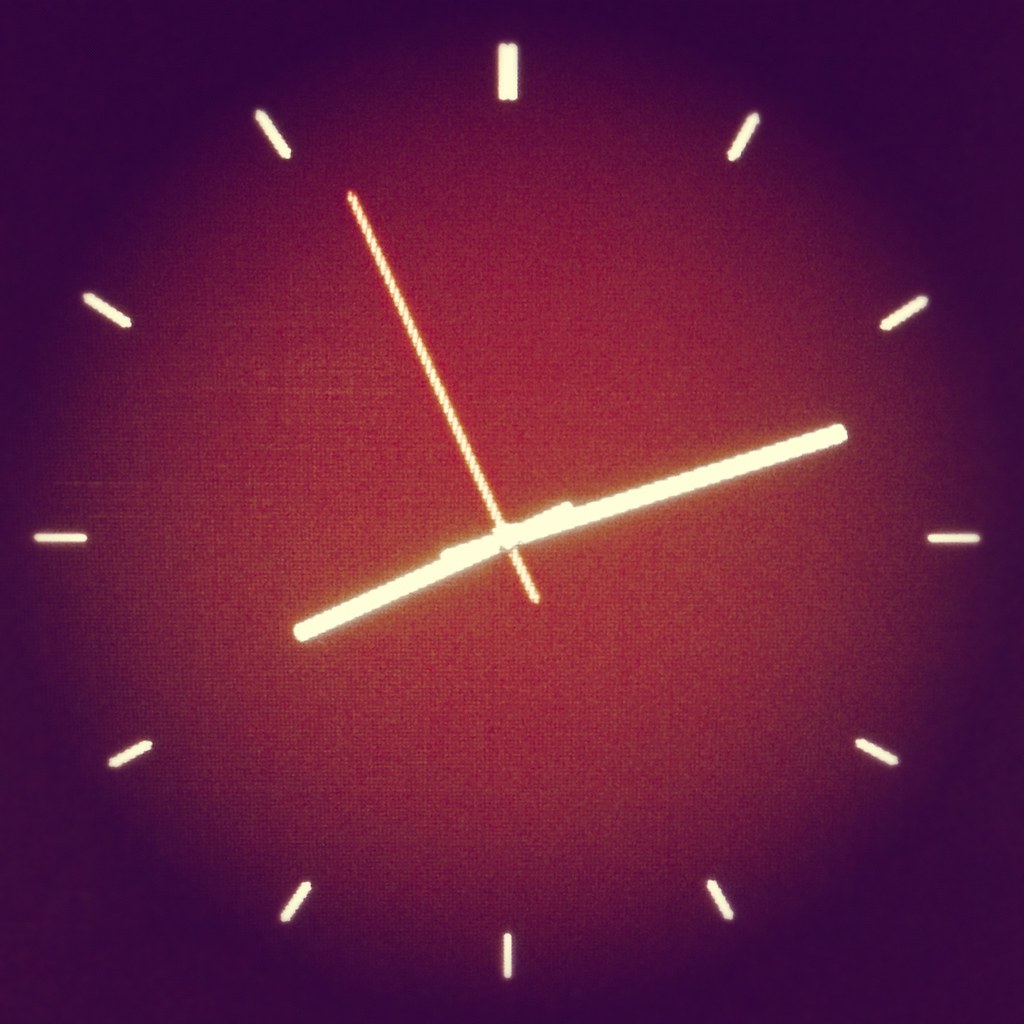The image features a stylized clock with no numbers, only hands and tick marks. The background is predominantly a deep purple, with a glowing red center. At the very center of this red hue is a small, pale yellow dot. Three clock hands extend from this dot: a short hour hand, a longer minute hand, and a slender second hand. Surrounding the transition from red to purple are dashes indicating where numbers would typically be on a clock face. Although numerical indicators are absent, the hands suggest the time is approximately 8:17.